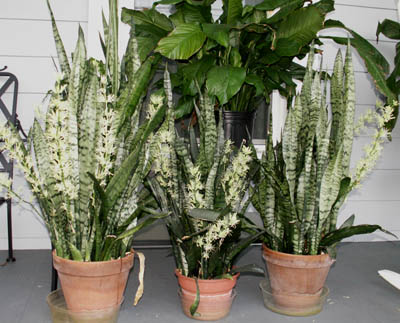The photograph features a cozy porch scene with four potted plants prominently displayed. In the forefront, three reddish-brown clay pots house a mix of plants with tall, slender blade-like leaves that are green with white stripes, interspersed with flowering stems showcasing delicate white blooms. These diverse plants share their space harmoniously, their fronds turned to reveal their undersides. Behind them, perched on a shelf, is a larger plant with expansive, umbrella-like green leaves growing from a black plastic pot. The background reveals white wood paneling indicative of a home's exterior, with a storm door barely visible in the middle. A hint of a chair with black iron details peeks in from the left, while the leg of a white object, possibly a rocking chair, is visible in the bottom right corner. The scene rests upon a gray concrete porch, adding a touch of rustic charm to the arrangement.